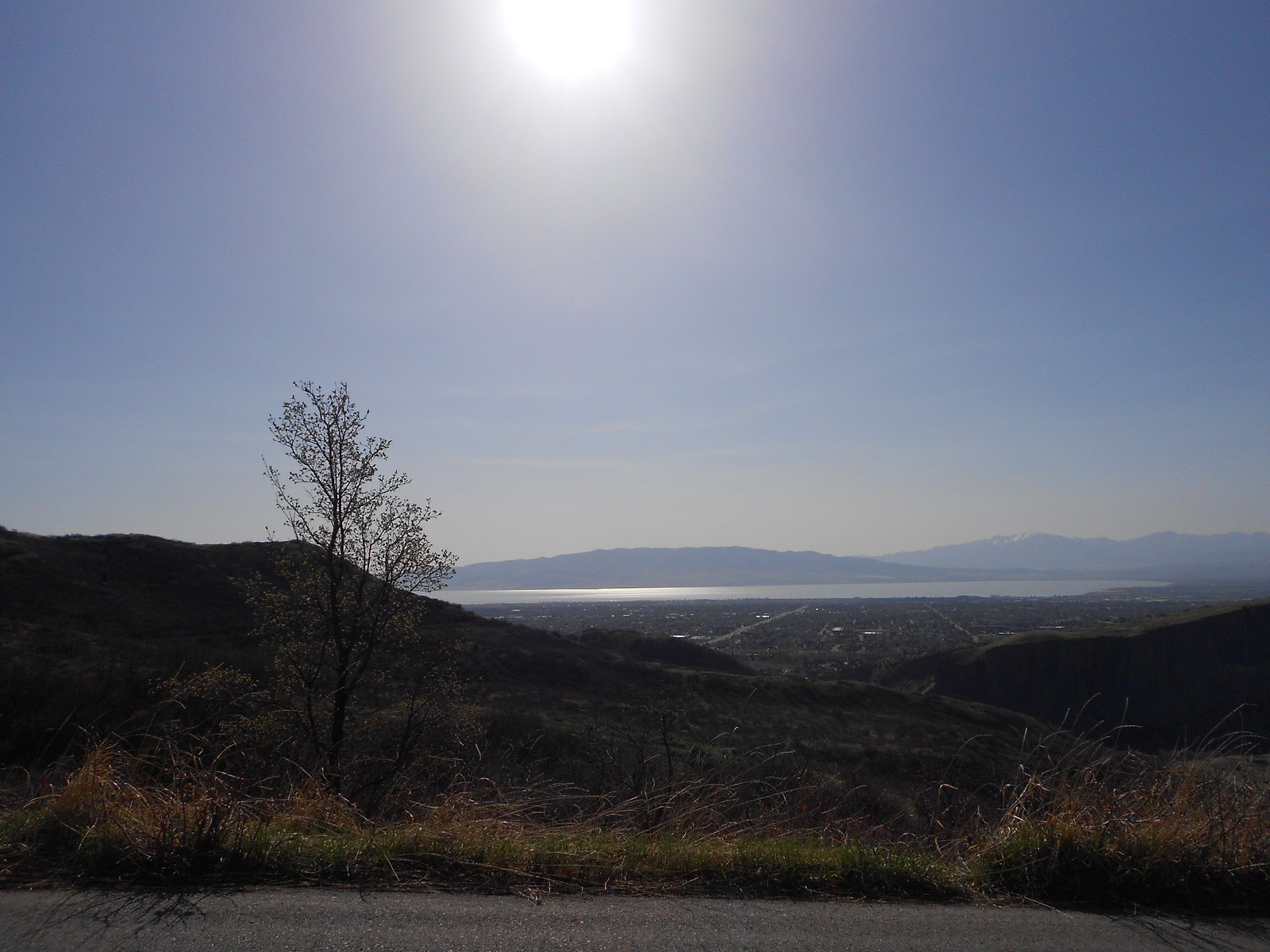The image captures a stunning aerial view of a sprawling landscape at sunset. Set against a clear blue sky with a bright, white sun descending towards the horizon, the scene showcases a diverse terrain. In the foreground, dark dirt hills are adorned with sparse, hay-like dead leaves, shrubs, and a lone, leafless tree with bare brown branches, indicating a fall season. Further into the distance, the landscape transitions into a larger field of grassy, rolling hills. Beyond these hills lies a cityscape, with visible roads winding through it. The city is bordered by a vast body of water, possibly a lake or bay, reflecting the sun's glow. On the far side of this water, majestic mountains rise, completing the picturesque vista.